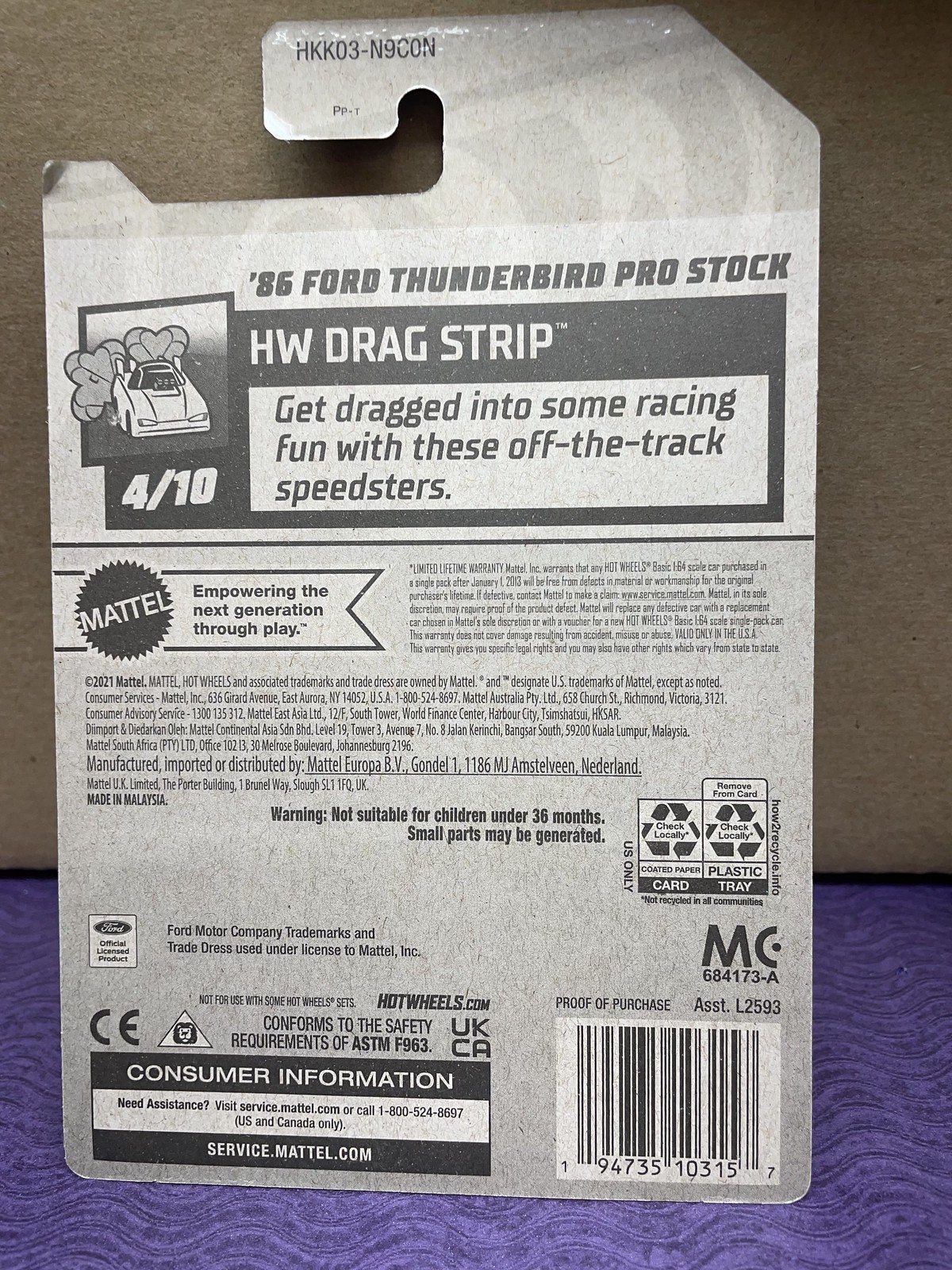The back of the package for a Hot Wheels car, specifically the "86 Ford Thunderbird Pro Stock", is photographed sitting on a purple wavy-textured carpet with a tan fabric background that resembles a couch. The packaging, intended to be hung on a peg hook, features a rectangular shape with a hook at the top. The text on the packaging includes multiple pieces of information in black lettering. At the top, it states "HKK03-9CON", followed by the car name "86 Ford Thunderbird Pro Stock" and "HW Dragstrip". 

It encourages enthusiasts to "Get dragged into some racing fun with these off-the-track speedsters", and mentions "4 out of 10", hinting at a possible collectible series. The text continues with a detailed description of the limited lifetime warranty by Mattel Inc., assuring buyers that any Hot Wheels Basic 1:64 scale car bought as a single pack after January 1, 2013, will be free from material and workmanship defects. 

Additional information includes a warning that the toy is "not suitable for children under 36 months" due to small parts. There's a mention of recycling details for the card and tray, and legal information about Ford Motor Company trademarks used under Mattel's license. Consumer support details are provided, directing users to service.mattel.com or a contact number for assistance in the US and Canada. The bottom right side features the proof of purchase, a barcode (9473510315), and the web address hotwheels.com, indicating it was made available in the UK.